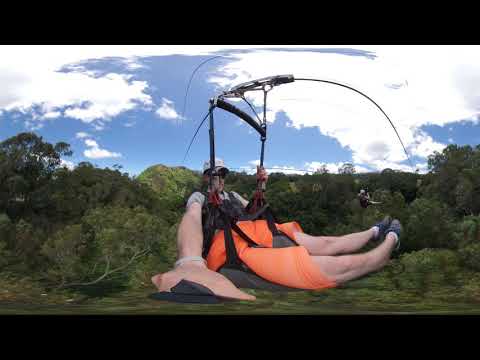The image depicts a man zip lining through a lush, green forest, captured in a highly distorted and exaggerated manner. The foreground shows the man with a dark helmet, gray shirt, and orange shorts, strapped securely with black harnesses to a cable. His legs are disproportionately large, especially the fat white thighs, due to the extreme distortion effect, which also affects his figure, making the closer parts look unnaturally big while the farther parts appear much smaller. One of his legs is oddly duplicated and enlarged behind him. He is possibly holding a tool or taking a selfie, adding to the chaotic composition. The background features a vibrant mix of green trees, blue sky, and white clouds, though the destination of the zip line is cut off from the frame. The overall scene is accentuated by horizontal black stripes on the top and bottom, emphasizing the vertical rectangular shape of the image.